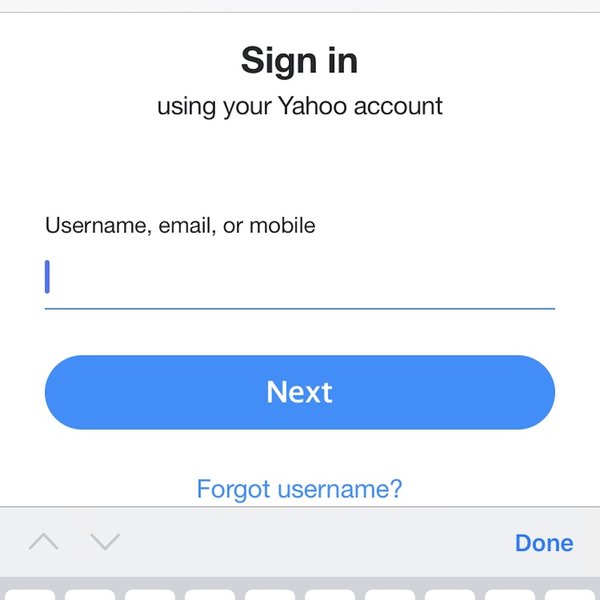The image depicts a sign-in screen for Yahoo, sized slightly wider than a typical cell phone display. The screen features a mostly white background with the text "Sign in" prominently displayed in bold, large black font. Beneath this, in a smaller font, are the words "using your Yahoo account." Further down, there is some white space followed by the prompt "username, email, or mobile," written in smaller black text. 

Below this prompt, a blank line with a flashing cursor on the left side indicates where users can input their credentials. A blue cursor line is visible on the left of this input field. Beneath the entry field is a rectangular button with rounded edges, featuring the word "Next" in white text. Below this button is the text "Forgot username?" in blue font, which serves as a link.

Near the bottom of the screen, there is a partially visible gray box, indicating the top edge of an on-screen keyboard. This keyboard is a very light gray, with up and down arrows located on the left side and "Done" in bold blue text on the right. The gray box also reveals the tops of ten square keys with rounded edges, suggesting the presence of a virtual keyboard.